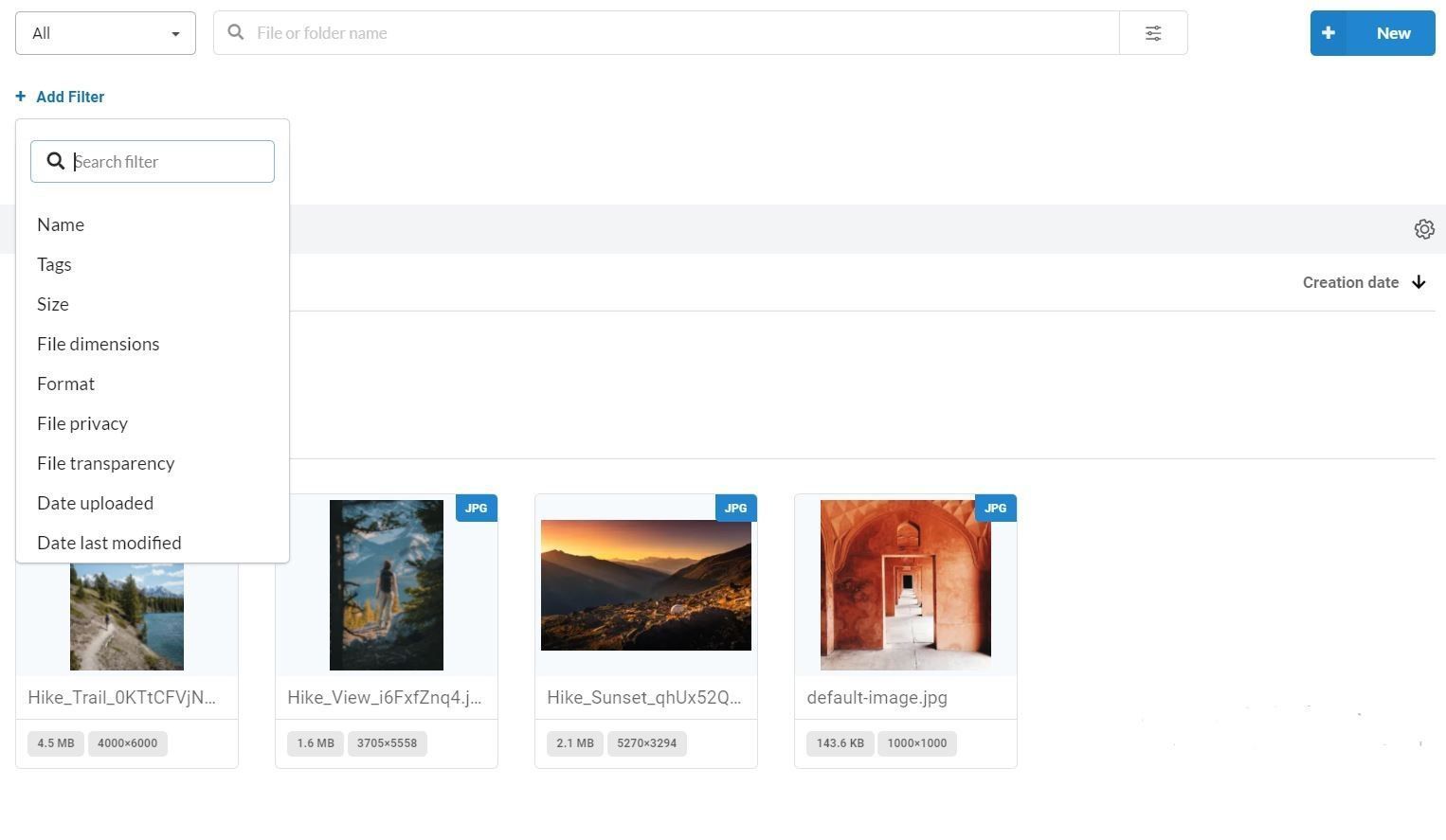This image is a detailed screenshot of a website interface with a white background. In the upper left corner, there is a dropdown menu labeled "Blackboard All" with a downward arrow icon indicating the menu can be expanded. Next to it is a search box featuring a magnifying glass icon, prompting users to search by 'file or folder name'. On the far right, there is a prominent blue button with a plus sign and the word "New" in white, suggesting the option to create or upload new content.

Below this top bar, on the left side, there is another blue button labeled "+ Add Filter," accompanied by an open dropdown list. This dropdown menu includes a search bar for filtering results further and below it, several filter criteria are listed in black text: Name, Tags, Size, File Dimensions, Format, File Privacy, File Transparency, Date Uploaded, and Date Last Modified.

A medium-sized gray bar spans across the interface beneath the filter section. On the far right of this bar is an icon resembling a flower head. Below, the words "Creation Date" appear with a downward arrow beside them, likely indicating sort options.

The main content area displays four image thumbnails in a grid format:
1. **"Hike Trail"**: Showcases a picturesque trail along a lake.
2. **"Hike View"**: Features a person overlooking a scenic view; this is a JPG file.
3. **"Hike at Sunset"**: Captures a sunset over a mountainous, semi-desert scene.
4. **"Default Image"**: Depicts the interior of a terracotta building, with a view through a series of doors revealing a tiled floor.

Each image thumbnail is accompanied by details of its file size and the amount of storage space it occupies in megabytes.